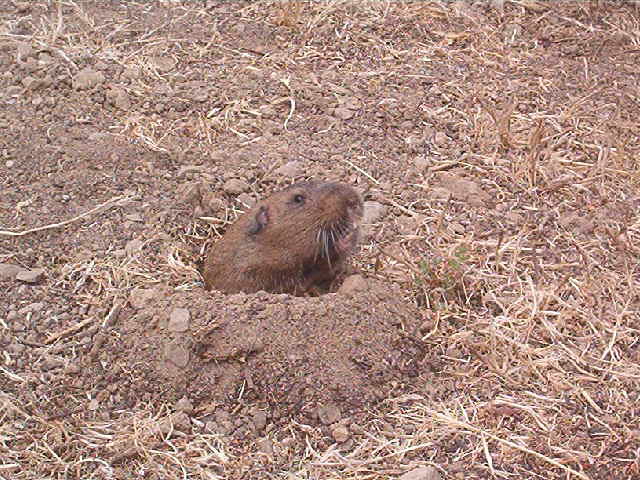In this detailed daytime image, a brown, furry gopher is emerging from a burrow in the ground, possibly freshly dug, creating a mound of dirt around the entrance. The gopher's side profile reveals its dark eyes, small ears, white whiskers, and prominent front teeth, with its mouth appearing slightly open. Dried, overgrown grass and scattered weeds mix with the predominantly dirt terrain, hinting at a hot and arid environment. One can also notice clumps of dirt in the upper left corner of the image. The overall impression is of a curious rodent cautiously surveying its surroundings from its earthy refuge.